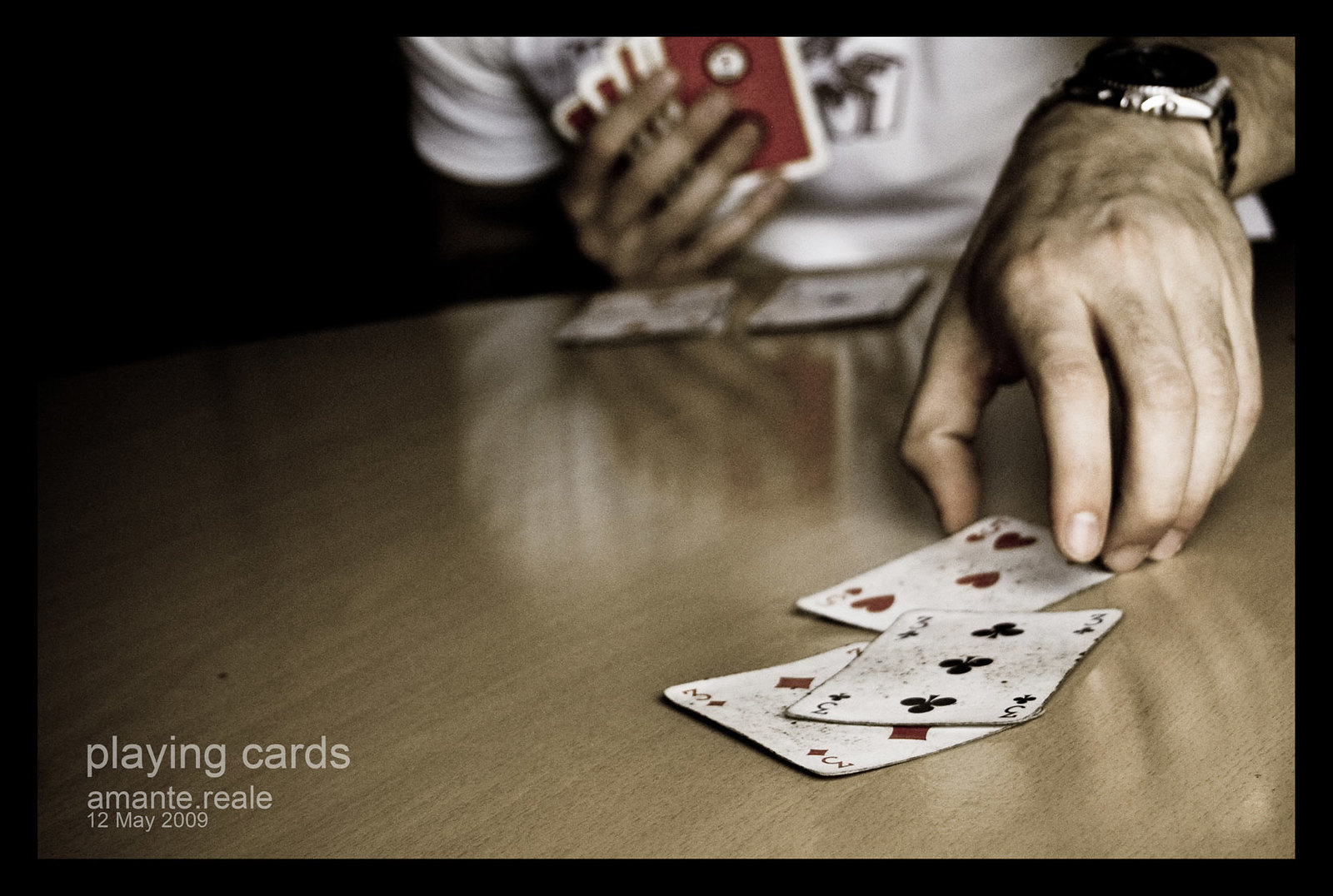In this image, a man is engaged in a game of cards, though only the lower portion of his body is visible. The frame extends up to his mid-torso, cutting off just before his chest. He holds a hand of cards in his right hand while his left hand reaches for the five of hearts card on a brown table. His attire includes a white, long-sleeved shirt and a silver metal watch on his left wrist. 

Three cards are visible on the table: the five of hearts, the three of spades, and the three of diamonds. Additionally, there are two small stacks of cards placed in front of him. The bottom left corner of the image contains the text "playing cards," followed by the name "Amante.Rielle" and the date "12 May 2009." 

The setting appears to be a dimly lit room, enhancing the focus on the man, his hands, and the cards. The left side of the image is largely obscured by shadows. The photograph carries a grainy texture and has a slightly desaturated color palette, indicative of its age and the date mentioned.